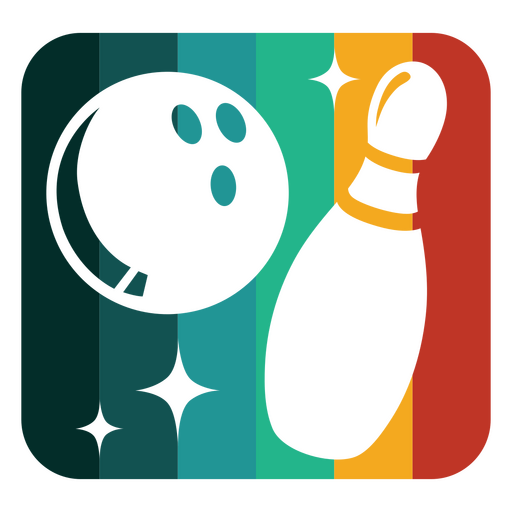This image is an animated, pop-art-style graphic of a bowling ball and a bowling pin set against a colorful background of six vertical stripes. The square image with rounded corners displays the stripes progressing from left to right as follows: a very dark green, an emerald green, a seafoam green, a turquoise, a mustard yellow, and a red. The white bowling pin is positioned diagonally, with its top in the top right corner and its base toward the middle of the image, while the white bowling ball, featuring three finger holes, is situated in the upper left-hand corner. Additionally, three small white diamond shapes or star-like sparkles are arranged around the ball and pin, enhancing the pop-art aesthetic.